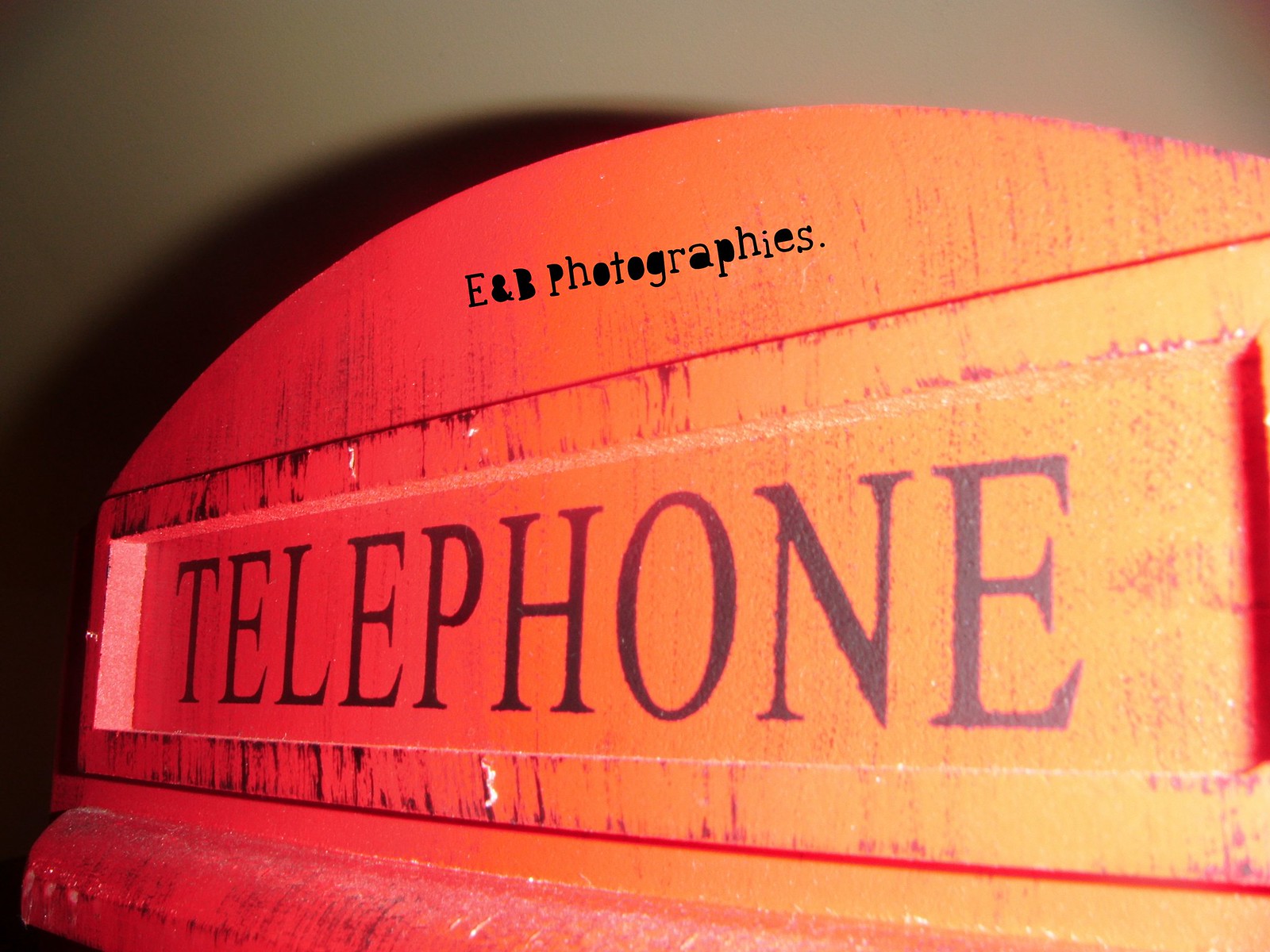The image depicts the top section of an old-school British telephone booth, reminiscent of those often seen in movies or TV shows such as "Doctor Who." The iconic design features a rounded, red top, a hallmark of classic British telecommunication. Below the curved roof, the structure transitions into a more rectangular form with a slight curve at the bottom. A rectangular framed area houses the word "TELEPHONE" in an all-caps, old-school font, printed in black. Above this, the curved section bears the inscription "E&B Photographies" in black lettering. The background consists of a light gray wall, with a shadow cast upon it by the top of the telephone booth, adding depth and contrast to the scene.